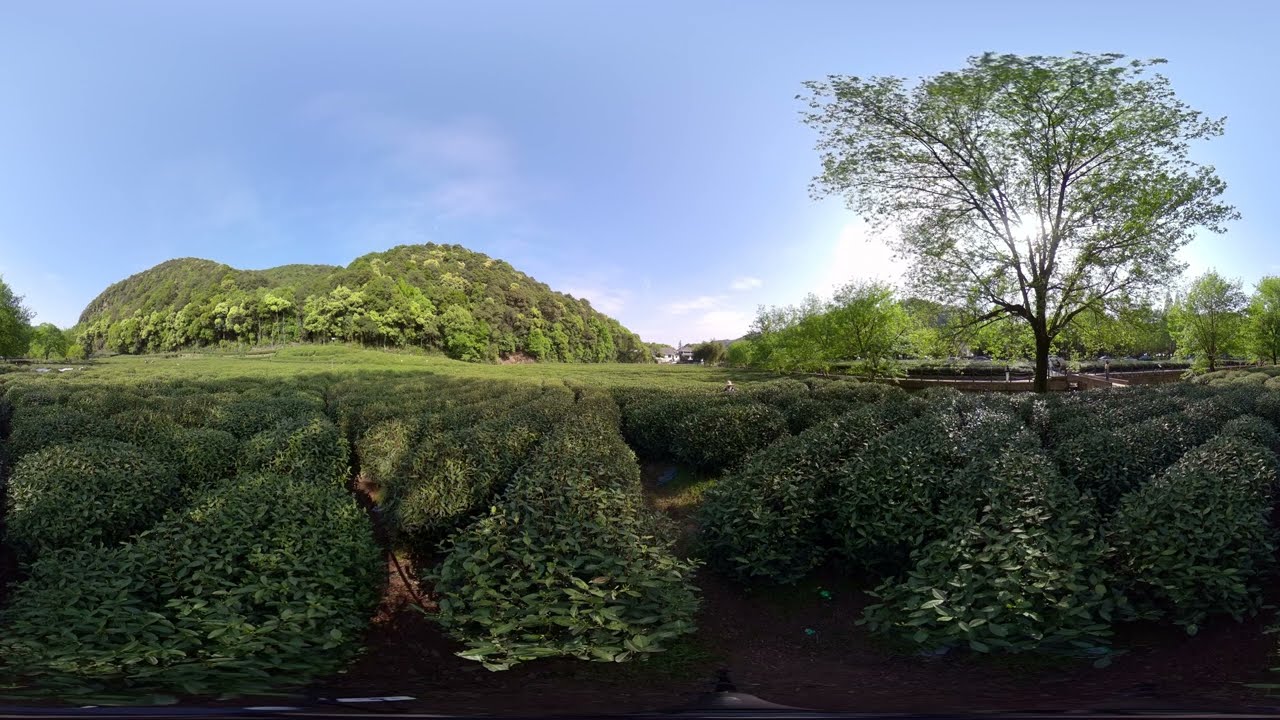The image portrays an outdoor scene characterized by a sloping landscape with a series of low hills and a valley in the center. The left part of the scene features a densely vegetated hill, while a slightly lower hill can be seen on the right side. The center of the image reveals a distant valley with indistinguishable structures that appear to be man-made. The foreground is rich with dense bushes, forming narrow paths through which one could walk, accompanied by visible patches of dirt and dark areas beneath the dense foliage. 

On the right side of the frame stands a large, sparsely-branched tree with the sun partially visible behind it, casting light that creates a contrast against the tree’s silhouette. The sky above is predominantly blue with sparse clouds. Below the main tree on the right, there is wood fencing, adding an element of human presence within the natural landscape. 

The entire scene is bathed in daylight, allowing the various earthy tones — greens of the vegetation, browns of the dirt, and the off-whites of the clouds — to be vividly captured.